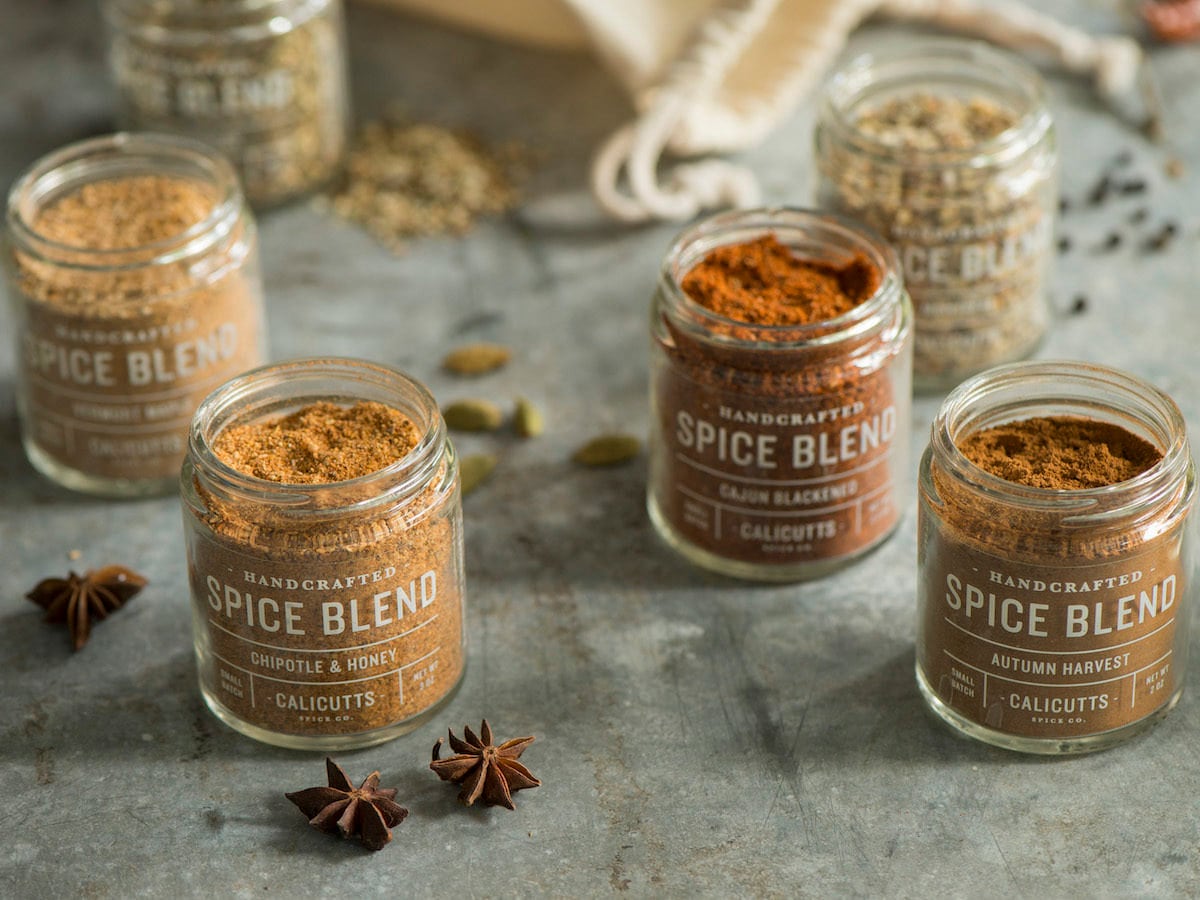This detailed color photo captures a close-up of six small, round mason jars filled with handcrafted spice blends, displayed on a gray felt surface. The jars are arranged in a row with their lids off, showcasing a variety of powdered spices in shades of sand, burnt orange, white, and medium orange. The labels on three jars are clearly legible: "Chipotle & Honey," "Cajun Blackened," and "Autumn Harvest," each marked with "Cow Cuts." The other three jars are partially blurred, but still reveal that they contain similar spice blends. Scattered around the jars are various spice elements, including star anise, adding to the rich, aromatic aesthetic. In the background, a beige drawstring bag with a white interior is slightly blurred, emphasizing the focus on the spice jars. The ambient lighting casts subtle shadows on the jars, enhancing the depth and warmth of the image. The overall scene suggests an advertisement for a gourmet spice collection.